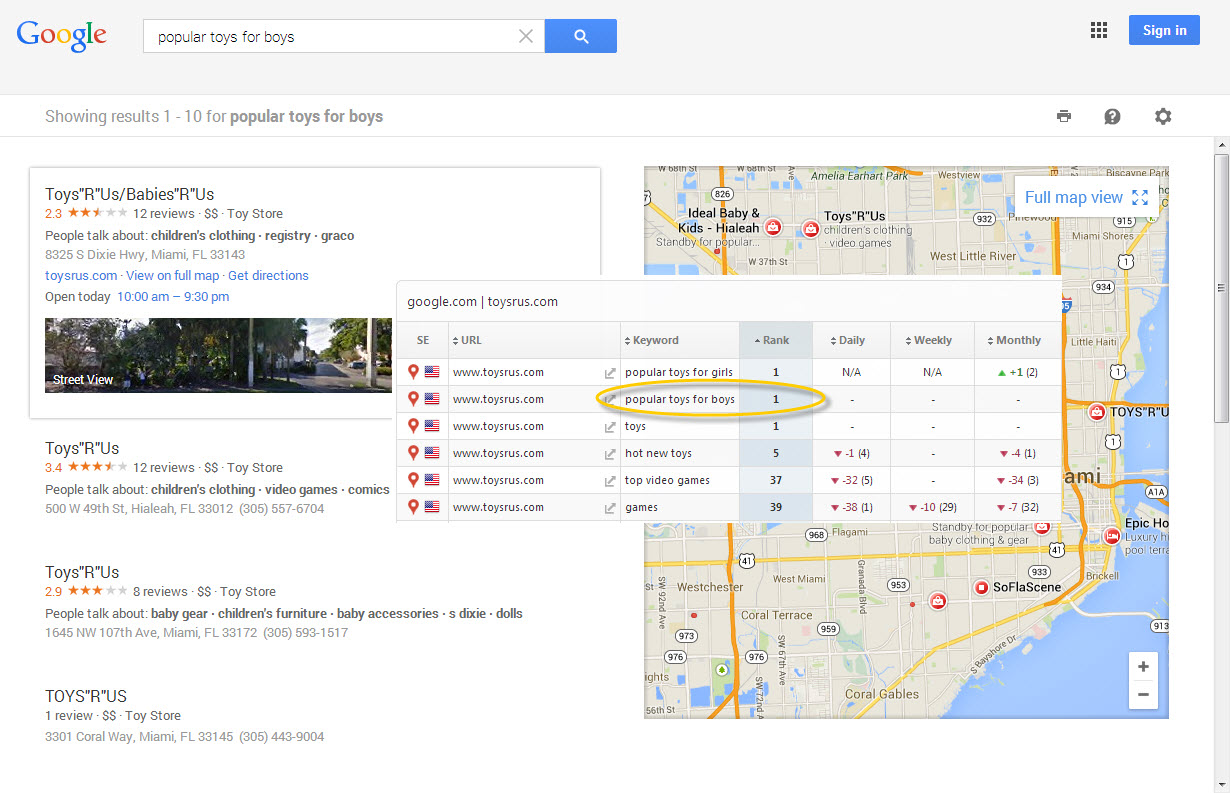The image showcases a Google search results page. At the top of the screen, there is a gray bar, which leads to the iconic colorful Google logo (blue, red, yellow, and green) situated on the left. The search bar contains the query "popular toys for boys," along with a small 'X' to clear the text and a blue search button with a magnifying glass icon on its right side. Further to the right, there is a grid icon formed by nine squares, and next to it, a blue "Sign in" button with white text.

Below this header section, the left side of the screen indicates that it displays "showing results one through ten for popular toys for boys." The left side lists various search results, while the right side features a map. Embedded within the middle of the screen is an SEO (Search Engine Optimization) analytics overlay that displays information about various URLs. It includes a header with columns labeled "SE," "URL," "Keywords," "Rank," "Daily," "Weekly," and "Monthly."

There are six rows of results beneath this header:

1. The first entry, identified by an American flag under "CE," is for toysrs.com with the keyword "popular toys for girls." It shows a rank 1 for daily, with figures "+1" and "2" in parentheses.
   
2. The second entry, which is highlighted with a yellow circle, relates to "popular toys for boys" under the same domain, toysrs.com. It has rank 1 daily, but the weekly and monthly stats are shown as "---."

3. The third entry again pertains to toysrs.com, simply marked as "toys." It shows no data for daily, weekly, or monthly.

4. The fourth listing is toysrs.hut, focusing on "new toys." It has a rank of 5, with daily changes noted as "-1" (with "4" in parentheses), no weekly data, and monthly changes showing "-4" (with "1" in parentheses).

5. The fifth entry is for "top video games," listed at rank 37, with a significant drop of "-32" daily (with "5" in parentheses), no weekly data, and a monthly drop of "-34" (with "3" in parentheses).

6. The last partially visible entry covers "games" without specifying any detailed data.